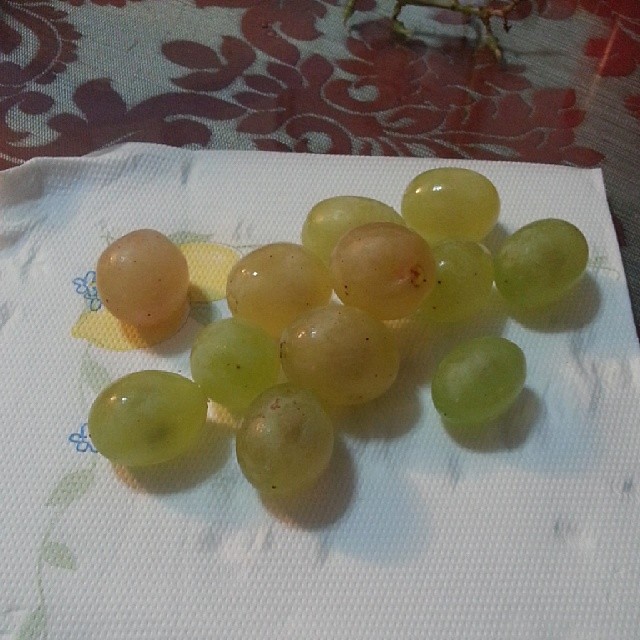The image portrays a dozen grapes scattered on a white napkin. These grapes vary from a lime green color to those tinged with purple; five of the grapes have notable purple tinting. Among them, two grapes display small black specks. The grapes, appearing plump and juicy, reflect the overhead light, enhancing their freshness and moist appearance. Some grapes are nestled together, while others are slightly apart or stacked. The napkin underneath features a decorative pattern on the top left corner, depicting two lemons with a blue flower and a green leaf. This napkin rests on a gray table adorned with red designs resembling the fleur-de-lis. In the top right corner, a portion of an object with a red base is partially visible.